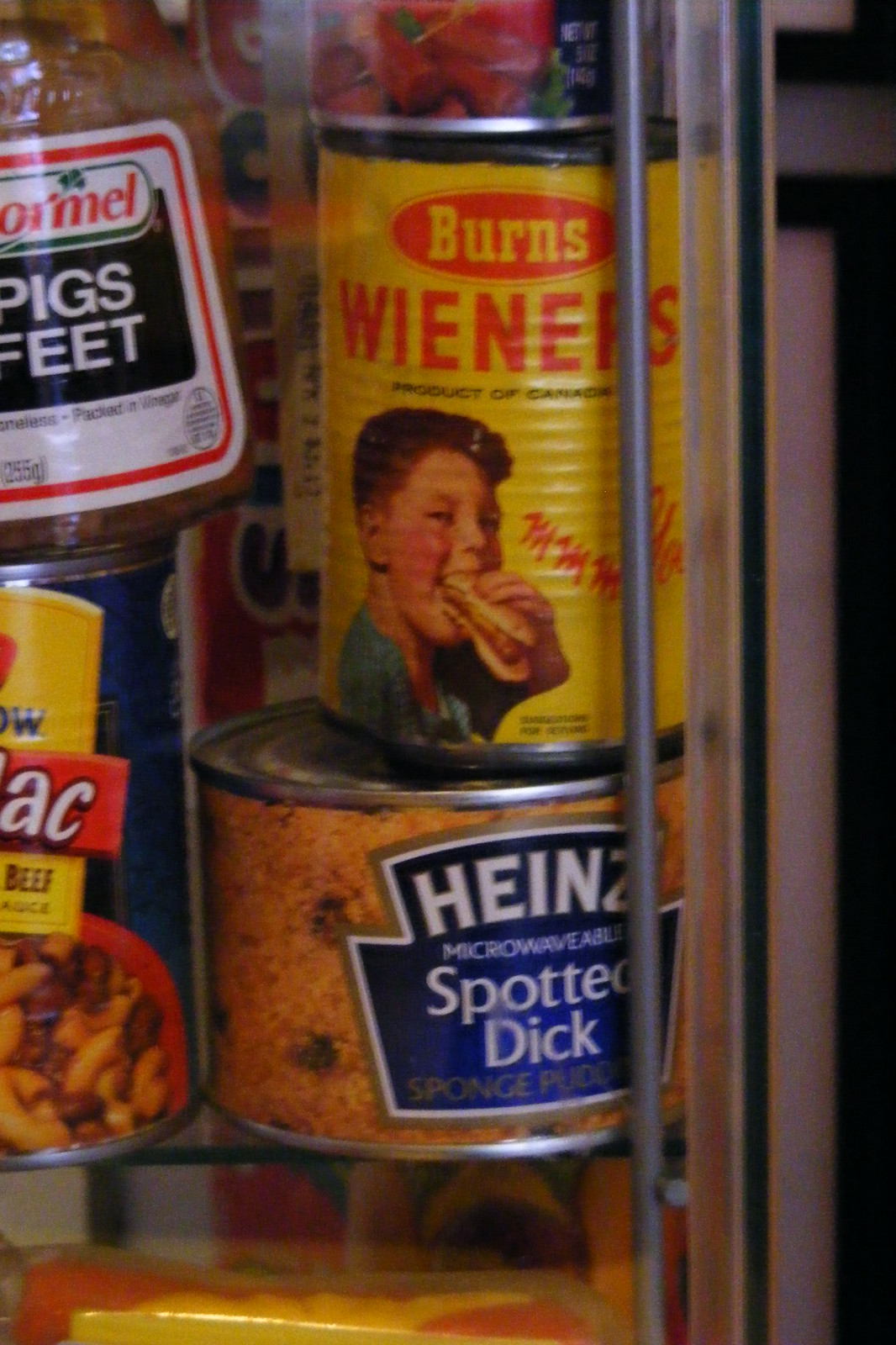This image, seemingly captured in an old pantry, showcases a nostalgic collection of vintage canned goods likely dating back to the 1970s or earlier. The focal point at the bottom is a small, double-tuna-sized can of Heinz Microwavable Spotted Dick, a sponge pudding, featuring a blue label with white lettering. Just above it, there is a vibrant yellow can with red lettering, labeled Burns Wieners, a product of Canada. The can sports an illustration of a cheerful, rosy-cheeked boy wearing a green t-shirt and enthusiastically munching on a hot dog.

To the left of the Burns Wieners can sits a Hormel Pigs Feet container, a curious reminder of past culinary preferences. Adjacent to the Heinz can, there appears to be a can resembling beefaroni, showing the partial text "AC Mac" on a blue label, indicating macaroni with beef. The incomplete label also features yellow and red elements. This collection of retro cans evokes a sense of culinary history and the diverse array of preserved foods that were once kitchen staples.